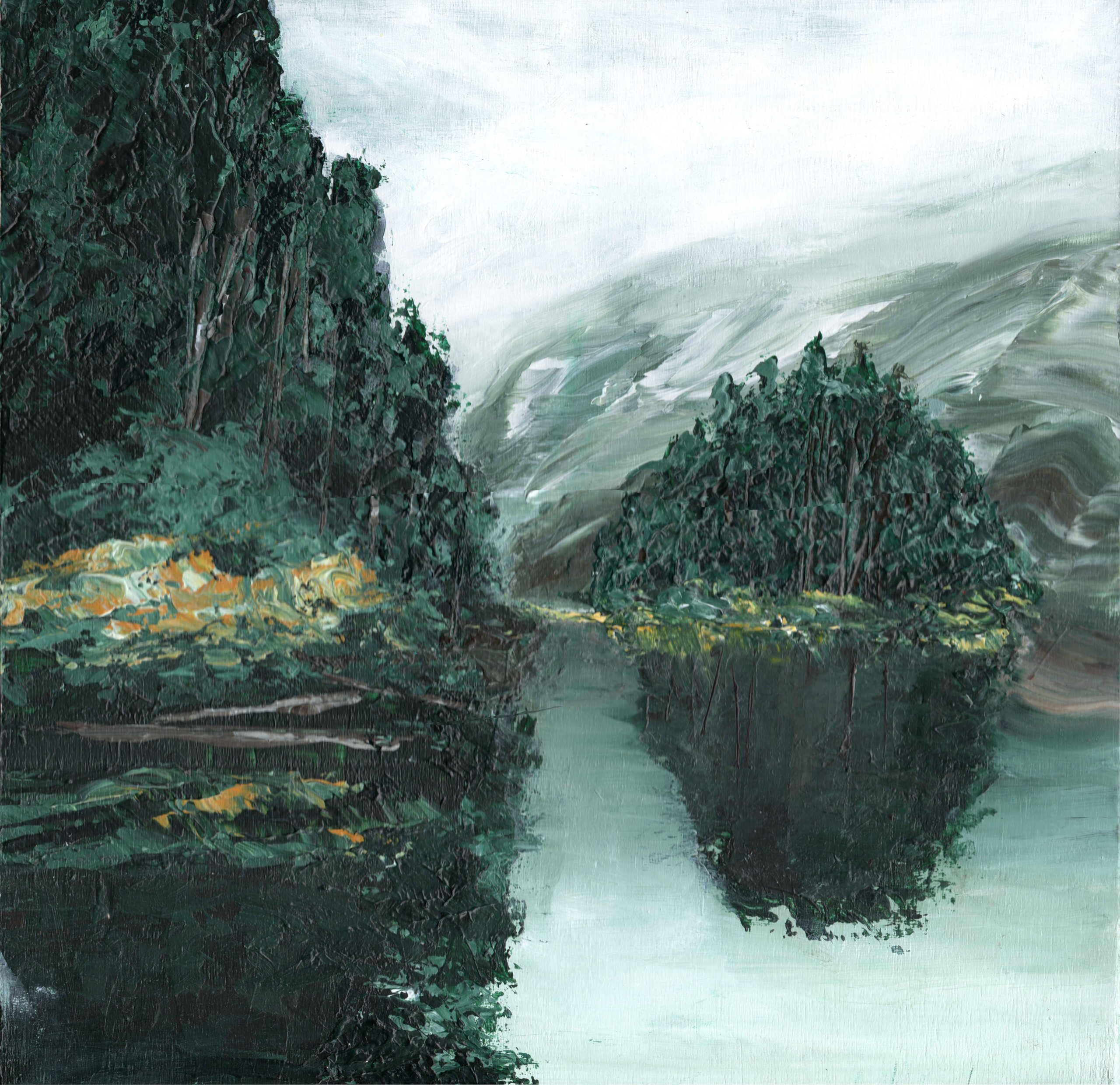This watercolor painting captures a serene lakeside scene with a dense forest and distant mountains. On the right-hand side, tall, closely packed trees extend toward the middle of the composition, their reflections mirrored perfectly in the water below. These reflected trees and grasses create an almost symmetrical, calming effect on the bottom left-hand corner of the painting. The water itself is mostly a light blue, intermixed with shades of gray and white, suggesting a tranquil, reflective surface. Beyond the trees, hints of a mountain range are visible, rendered in blended shades of green and white. The sky above is cloudy, predominantly white with touches of light gray and subtle hints of blue, enhancing the dreamy atmosphere. To the left of the painting, more tall trees and thick vegetation are seen, with colorful bushes that include hues of yellow, all reflected in the lake's serene waters.